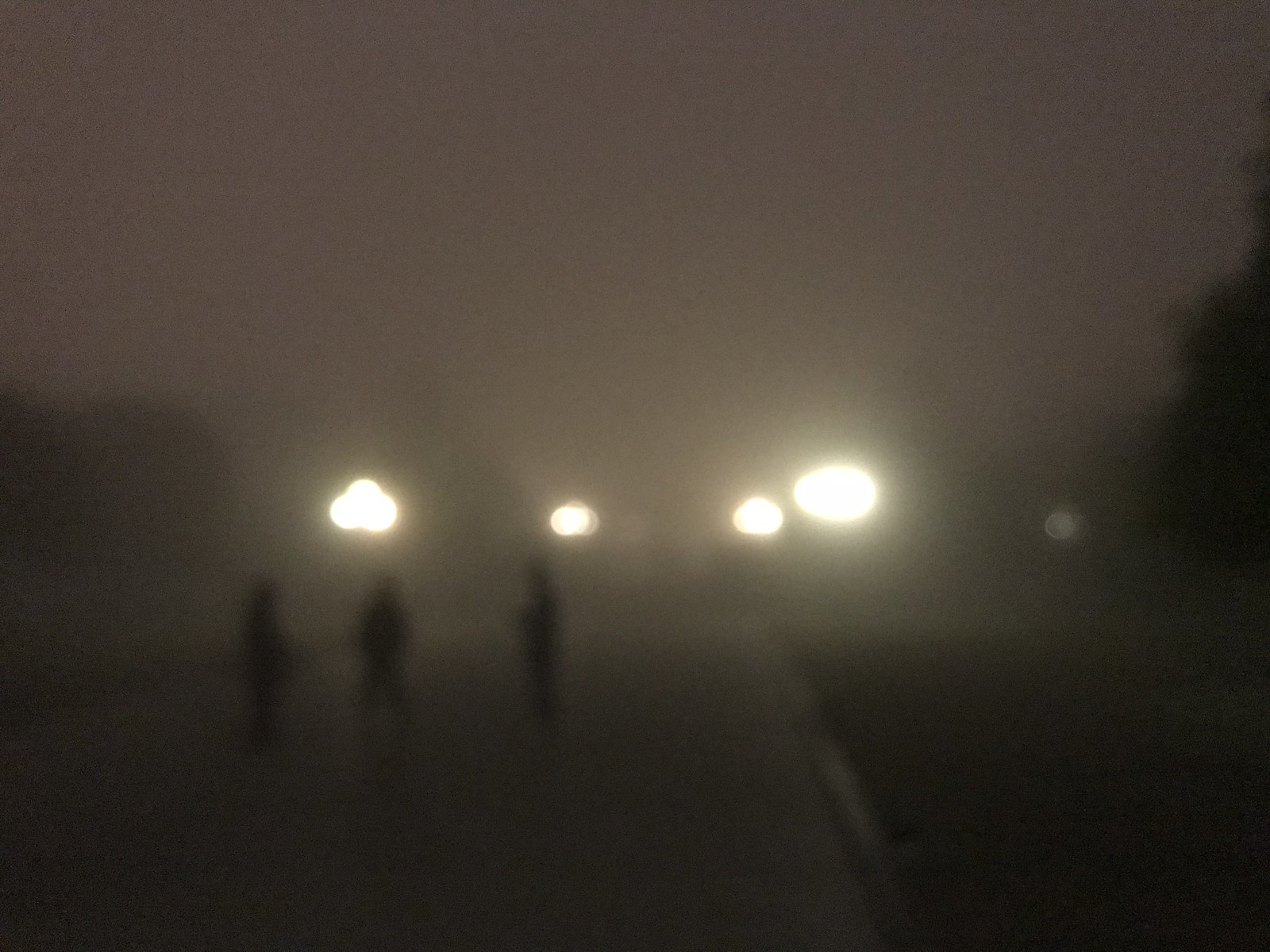The photograph captures a nighttime outdoor scene shrouded in a thick layer of fog and haze, rendering the image very blurred. The sky has a grayish-red tint, adding a surreal quality to the atmosphere. In the distance, four street lights glow faintly, casting a dim light on the surroundings. Flanking the scene on both sides are trees, with a grassy area visible to the left side of the image and a paved pathway or street running through the center. Toward the bottom left of the photograph, three silhouetted figures are standing together, seemingly engaged in conversation. Due to the heavy fog, their features are indistinguishable, appearing only as dark, shadowy shapes.